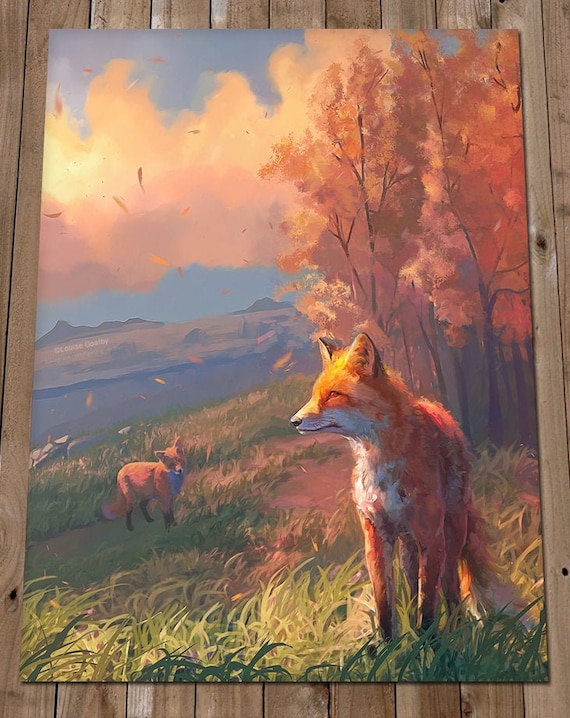This painting, displayed on a medium brown paneled wall with vertical lines, depicts a vibrant natural scene featuring two foxes. The foxes, characterized by their orange fur, white underbellies, and white markings around their mouths and throats, are positioned in a grassy area. The fox in the foreground, situated towards the right side of the painting, faces the viewer, highlighting its bushy tail, almond-shaped eyes, and the sun's light reflecting off its head. Surrounding this fox are tall trees adorned with orangish-red leaves, suggesting a fall setting. The other fox is positioned farther back in the field. The backdrop showcases majestic mountains and an expansive sky adorned with puffy white clouds tinged with a pinkish-orange hue. This harmonious blend of orange hues in the foxes, trees, and the sky creates a vivid and breathtaking autumnal landscape.